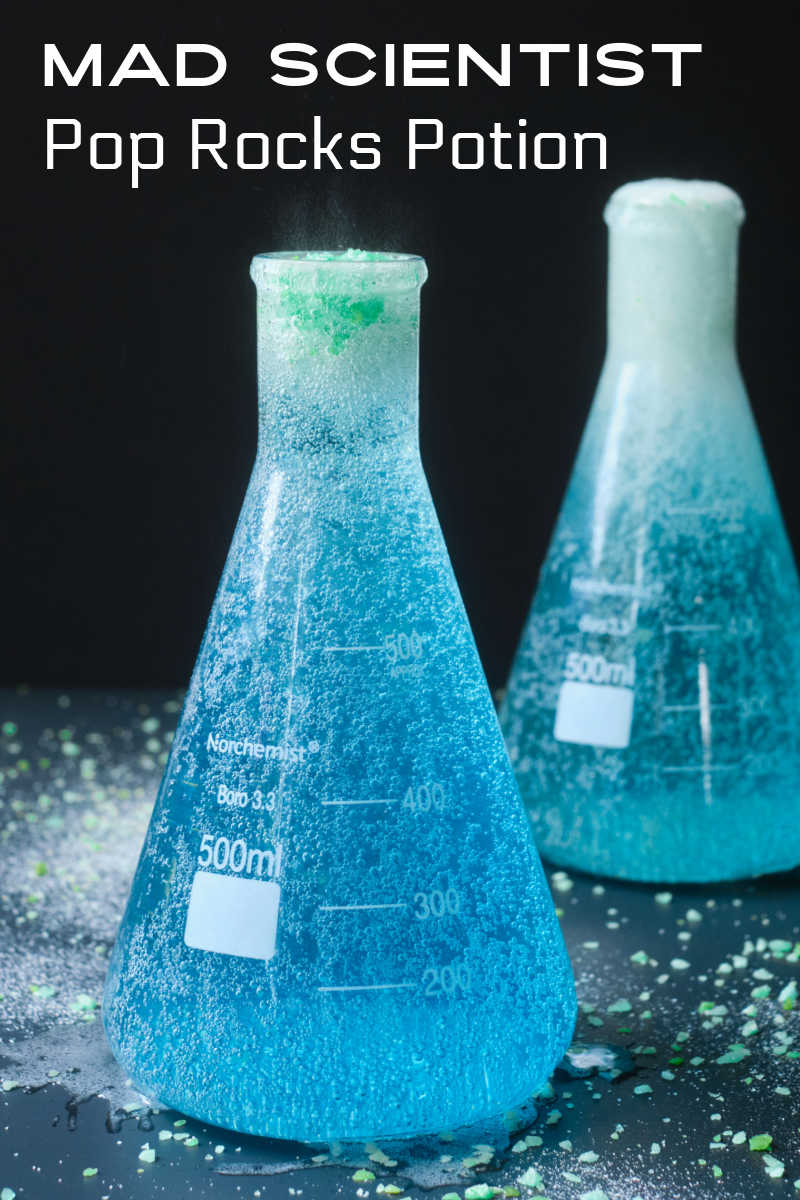This rectangular photograph, measuring approximately six inches high and three inches wide, depicts two scientific beakers filled with a vibrant turquoise-blue liquid, creating an executed scene under the theme 'Mad Scientist Pop Rocks Potion’. The phrase "MAD SCIENTIST" is prominently displayed in bold, all-caps white text at the top of the image, with "Pop Rocks Potion" written just below it, capitalizing only the first letters of each word.

Both beakers, labeled "Nor Chemist" and marked for a capacity of 500 milliliters, sit on a wet black table. Their contents are bubbling and fizzing dramatically due to the presence of colorful Pop Rocks candy—recognizable for emitting a popping sensation in the mouth when consumed. The measurement markings on the beakers start from 200 milliliters at the bottom and go up to 500 milliliters towards the top. One beaker, showing foam spilling out of its narrow opening, fades into a greenish hue at the top, whereas the other remains a consistent turquoise-blue with pale white at its upper edge. The table's surface is littered with scattered green and blue Pop Rocks alongside liquid spills, enhancing the experimental atmosphere.